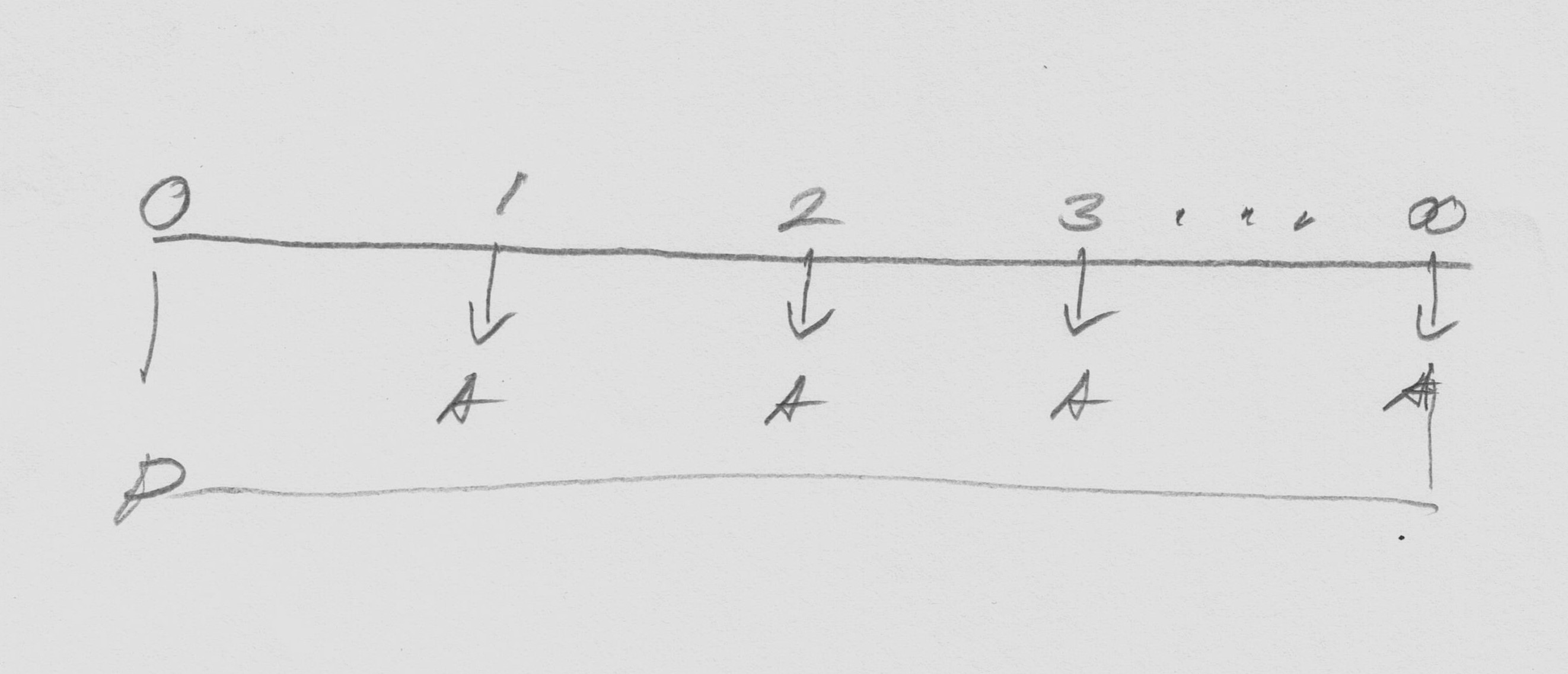This image depicts a hand-drawn graph created with a black pen or pencil on paper. The graph consists of a horizontal line marked with the numerals 0, 1, 2, 3, followed by an ellipsis (…). The series of numbers culminates in a symbol that appears to be an infinity sign, represented by two zeros placed side-by-side (∞).

Descending arrows are drawn from each number, directing towards the letter 'A' for each corresponding numeral. Below this main horizontal line, there is another line labeled with the capital letter 'P' at the beginning, stretching across the width of the graph. The overall appearance suggests an ordered illustration of a sequence or set, where every number is mapped to the letter 'A', and the entire assembly is underlined with a secondary line labeled 'P'.